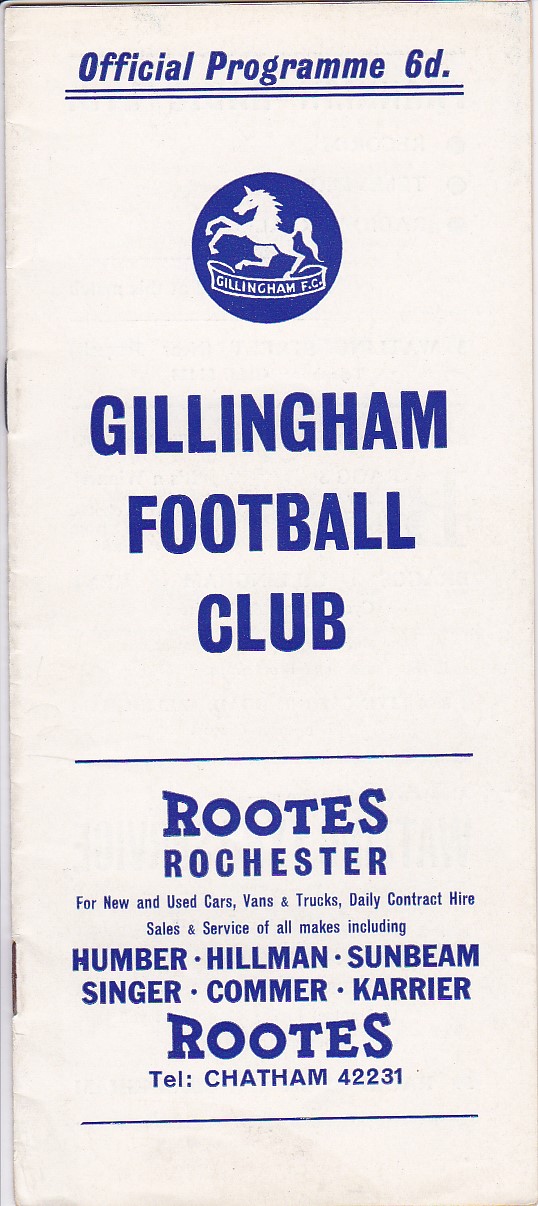This is a detailed color photograph of a tall, thin sports program, appearing to be stapled at two locations like a booklet. The program features a white background adorned with blue text. At the top, it reads "Official Program 6D" with blue underlines. Centered on the page is a blue and white logo, depicting a unicorn rising up on its hind legs within a blue circle, flanked by the text "Gillingham FC." Below this emblem, in prominent blue letters, it says "Gillingham Football Club." Beneath it is an advertisement for "Roots Rochester," promoting new and used cars, vans, and trucks, as well as daily contract hire, sales, and service for various makes including Humber, Hillman, Sunbeam, Singer, Commer, and Carrier. The contact number provided is "Telephone, Chatham 42231."